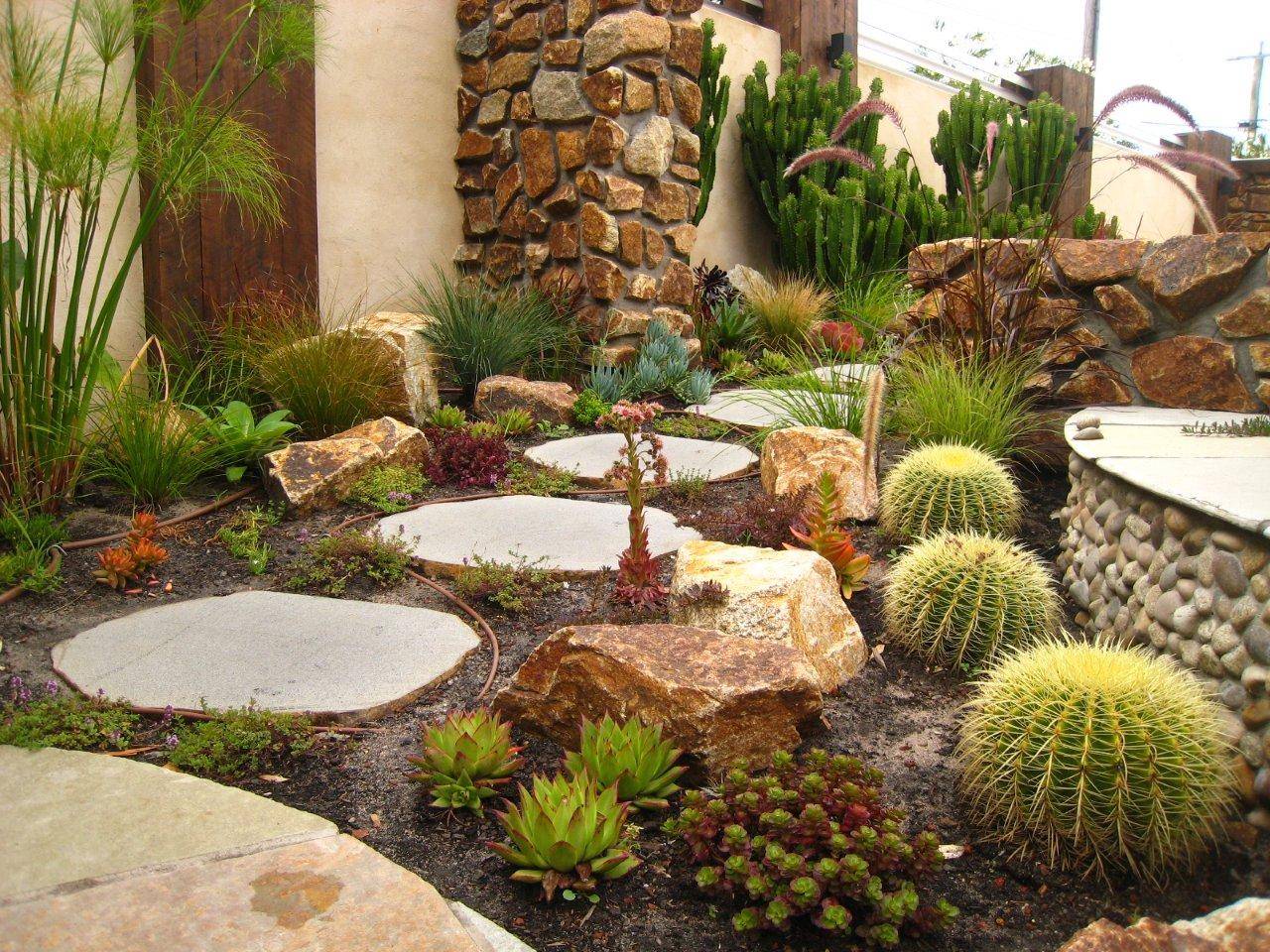The image depicts a garden, potentially part of a backyard or a botanical garden, meticulously organized with a variety of cacti and succulents. Dominating the scene is a pathway made from five large, flat, round stepping stones that traverse through an otherwise dirt landscape. To the right of the path, numerous cacti of different shapes, sizes, and colors are featured prominently, including some large, almost yellow, spiny cacti and smaller green varieties. The garden also includes stone structures and river stones, contributing to the architectural elements of the space. In the background, a power pole supporting electrical transmission lines is visible. The garden is bordered by an intricate masonry fence comprising stone pillars, wooden pillars, and stucco sections, giving a light-colored sandy appearance. There seems to be a terraced area made from rock and stone, intended for either seating or maintaining different elevations in the dirt. The detailed layout also hints at a secondary pathway in the bottom left corner, made from different stones.